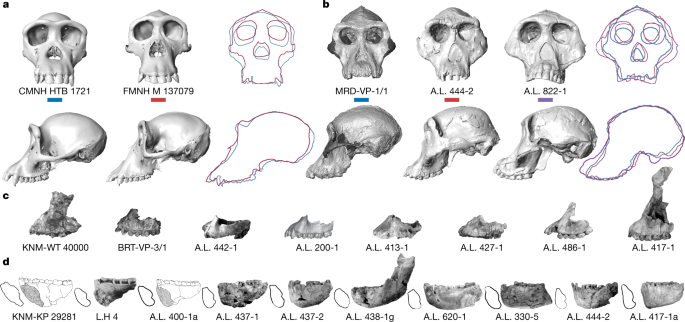This detailed chart features black-and-white illustrations and drawings of various skulls and bones arranged on a white background. There are four rows, with the top two rows displaying skulls and the bottom two rows depicting jawbones and other irregularly shaped bones. The first row consists of five frontal views of skulls and two drawn illustrations, showcasing detailed features such as foreheads, eye sockets, noses, and upper teeth. The second row presents side profiles of five skulls and two drawn illustrations. Each image is labeled with identifiers, such as CMNHHTB1721, FMNHM137079, and AL444-2 in the first row, and KNM-WT40000, AL427-1, and BRTVP3-1 in the second row. The bottom two rows highlight various bone fragments and jawbones, listed with labels like KNM-KP29281, LH4, and AL400-1A. These visual representations appear to be from the ape family, with some specimens displaying fangs. The chart provides a comprehensive array of skulls and bones, categorized and meticulously labeled for detailed study.